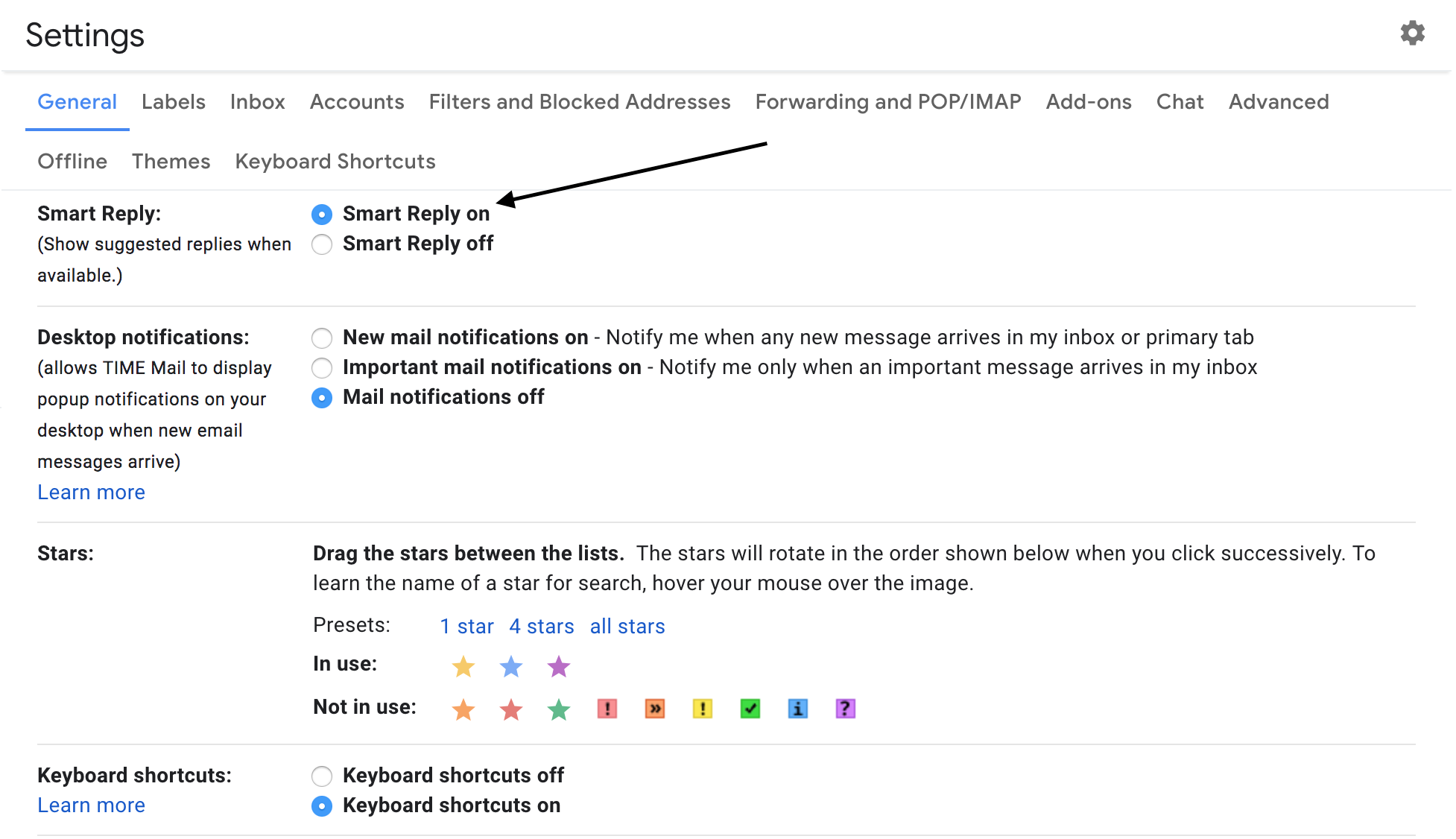This is a detailed screenshot of the Gmail Settings page, specifically highlighting the 'General' tab. At the top of the white webpage, it prominently displays the word "Settings." Below this header is a navigation bar with multiple tabs: 'General' (highlighted), 'Labels,' 'Inbox,' 'Accounts,' 'Filters and Blocked Addresses,' 'Forwarding and POP/IMAP,' 'Add-ons,' 'Chat,' and 'Advanced.' Beneath these primary tabs, there is another horizontal menu featuring 'Offline,' 'Themes,' and 'Keyboard Shortcuts,' although none of these options are selected.

Within the 'General' tab's interface, the setting titled "Smart Reply" comes first, offering an option to turn it on or off. The 'Smart Reply' feature has a blue dot next to the "On" option, indicating it is currently activated. An annotation arrow is pointing towards this setting, likely to guide users on how to enable or find "Smart Reply."

Following this section, the next setting is "Desktop Notifications." Here, users can choose between "New mail notifications on," "Important mail notifications on," and "Mail notifications off," with the "Mail notifications off" option currently selected.

Further down, there's a section for "Stars," which allows users to drag different colored stars between lists. These stars will then cycle in the order shown whenever clicked.

At the bottom of the page, the "Keyboard Shortcuts" setting is visible, with toggles for turning shortcuts on or off. The "Shortcuts on" option is highlighted, indicating that keyboard shortcuts are currently enabled.